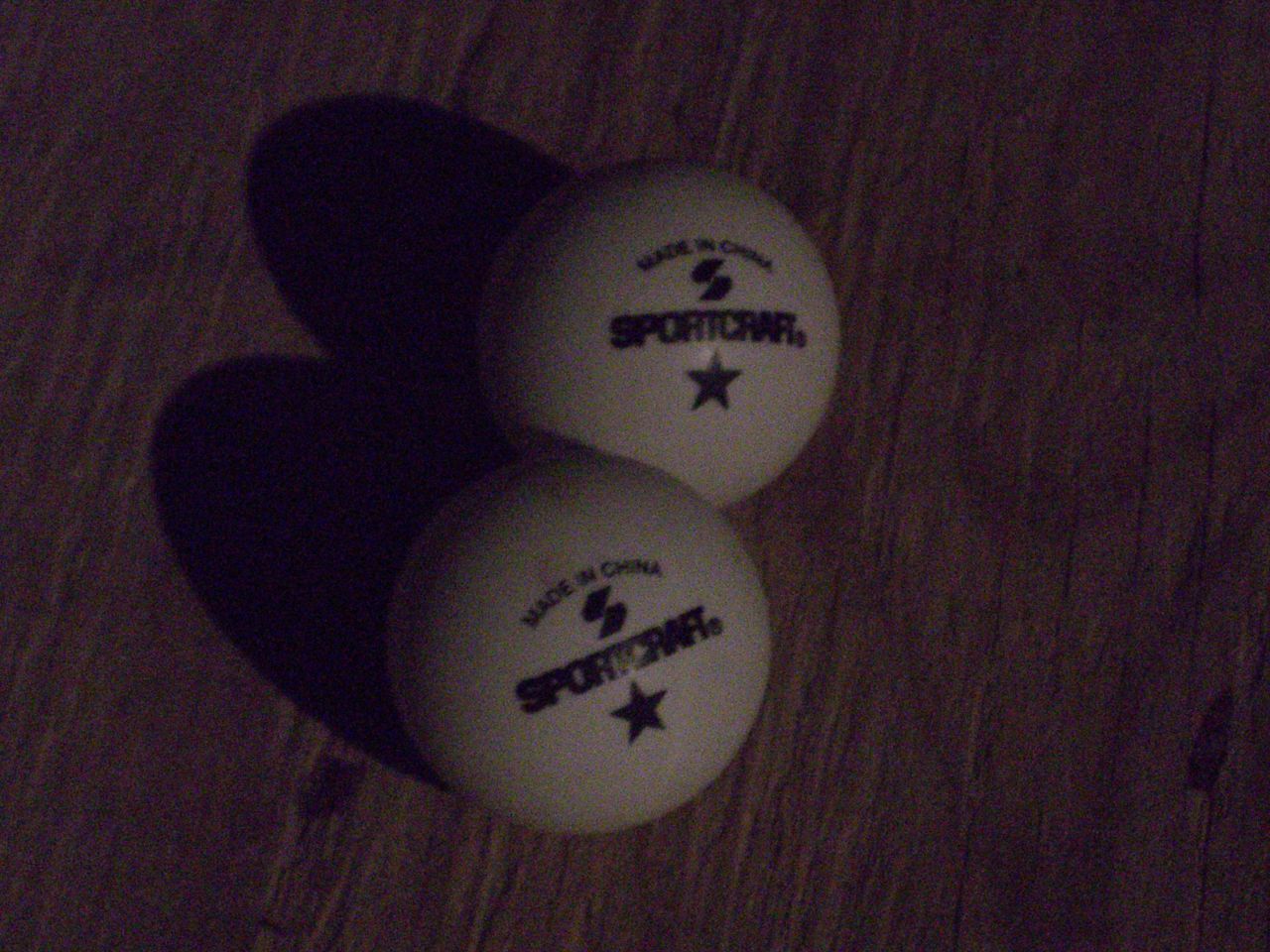In a dimly lit, grainy photograph, two white Sportcraft golf balls rest prominently on a rough wooden table surface. The focus is on the balls, which occupy roughly 30% of the image. Each golf ball bears the black text "Sportcraft" with a large black star beneath it and "Made in China" inscribed above, all centered amidst the visible wood grain of the table. The lighting, coming from the high right side, casts distinct shadows resembling eggshells behind each ball. The balls, aligned one above the other, display a glint of light reflecting off their surfaces, emphasizing their positioning and adding a subtle glow to the dark, rustic setting.